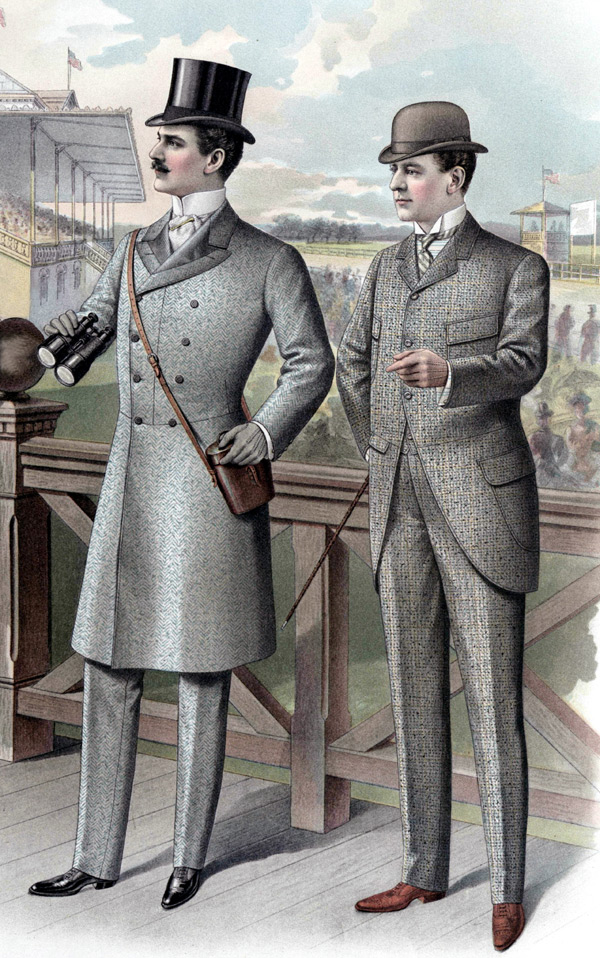This meticulously detailed artwork portrays two distinguished gentlemen from the late 1800s or early 1900s, presumably spectating at a horse or dog race. Situated against a sturdy brown wooden fence with crossbeam posts, the painting captures the lively atmosphere of the racetrack with the crowd in the stands and a cloudy sky looming above.

The gentleman on the left, adorned in a long gray coat, exudes elegance with his black top hat, dark hair, and neatly groomed mustache. He wears a high-necked, button-up white collar shirt beneath his coat and has a brown satchel slung across his shoulder, with his hand resting atop it. In his other hand, he holds a pair of binoculars, indicative of his interest in the race. His poised gaze is directed off to the left, and he is shod in impeccably polished black shoes.

His companion, slightly turned to the left and gesturing towards the same direction, is equally stylish in a brown derby hat. He wears a white collar shirt complemented by a striped tie, gray trousers, and brown shoes. The juxtaposition of their attire and their attentive stances against the picturesque backdrop vividly captures the essence of a race day from a bygone era.